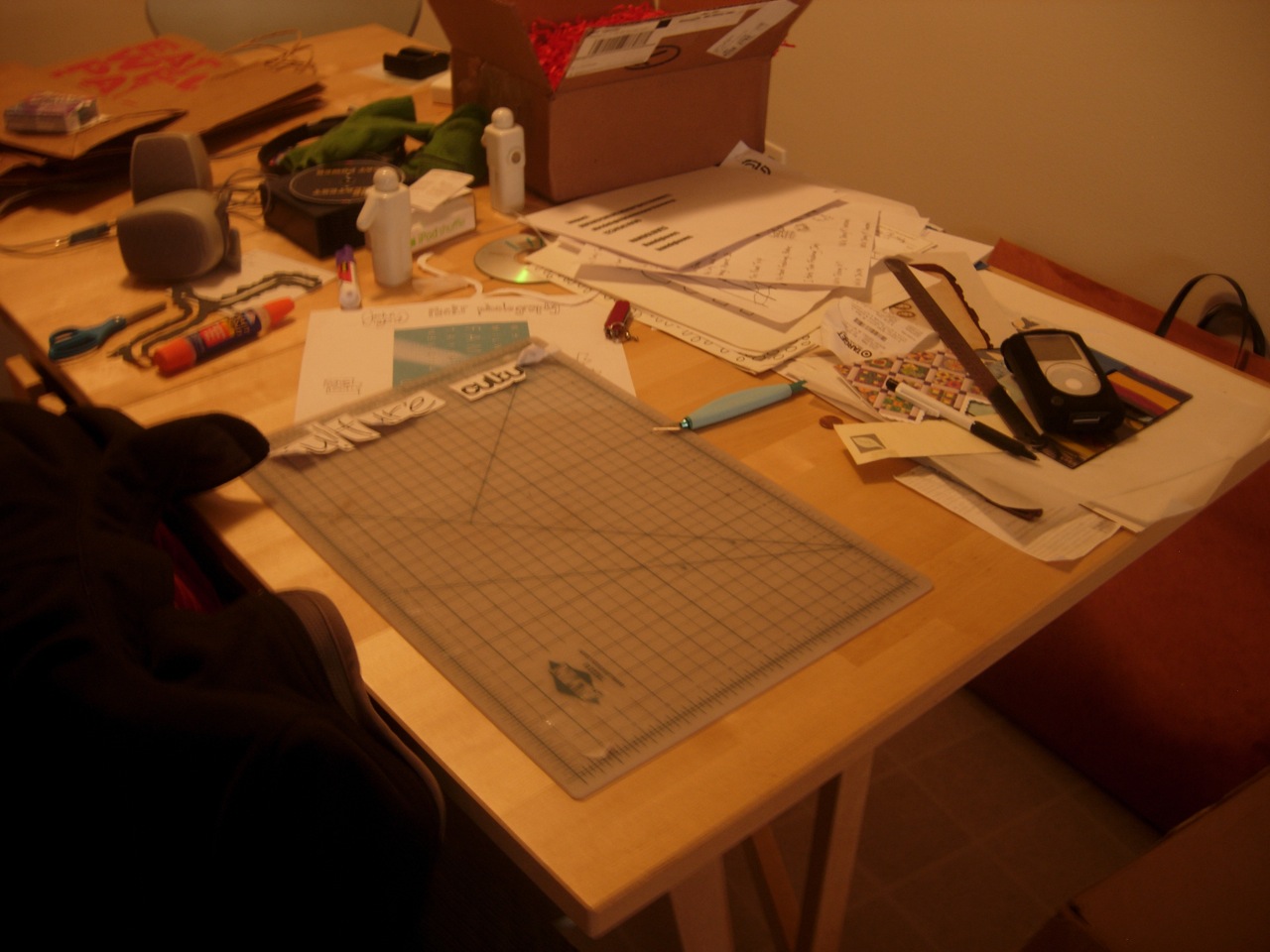The image depicts a heavily utilized work table, surrounded by red couches that provide seating. The white table surface is cluttered with a variety of tools and materials suggestive of frequent use, perhaps in a workshop or club setting. Among the items visible on the table are measurement tools resembling a thermometer, a box opener, various pens, and an unidentified tool. A grid map with letters and intersecting lines lies on the table, alongside several stacks of papers, one of which displays a bar chart. A cardboard box containing what appears to be plastic strips is also present. Additional items scattered across the table include a marker, scissors, a glue bottle, and a stapler. There is also a cardboard bag and a set of index cards towards the back. Two mysterious white cylindrical objects add to the miscellaneous assortment, making the table appear highly cluttered and indicative of ongoing projects or activities.